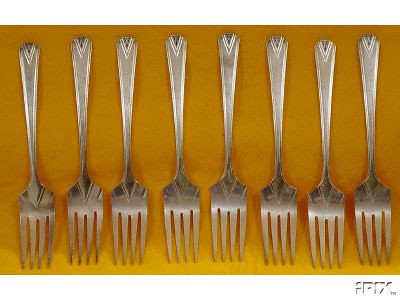This photograph features eight ornate silver forks aligned side by side, handles pointing upward against a yellow wall, which is also surrounded by a white border. The forks, made of what appears to be silver, showcase hints of black tarnish along the edges, indicating their age. They are standing on their tines, leaning against the wall, and reflecting bright light off their handles. The handles of the forks exhibit intricate, geometric designs, including triangular shapes near the tip and the base. In the bottom right corner of the image, there is a partially legible logo or watermark, possibly containing the letters F, P, I, and X.